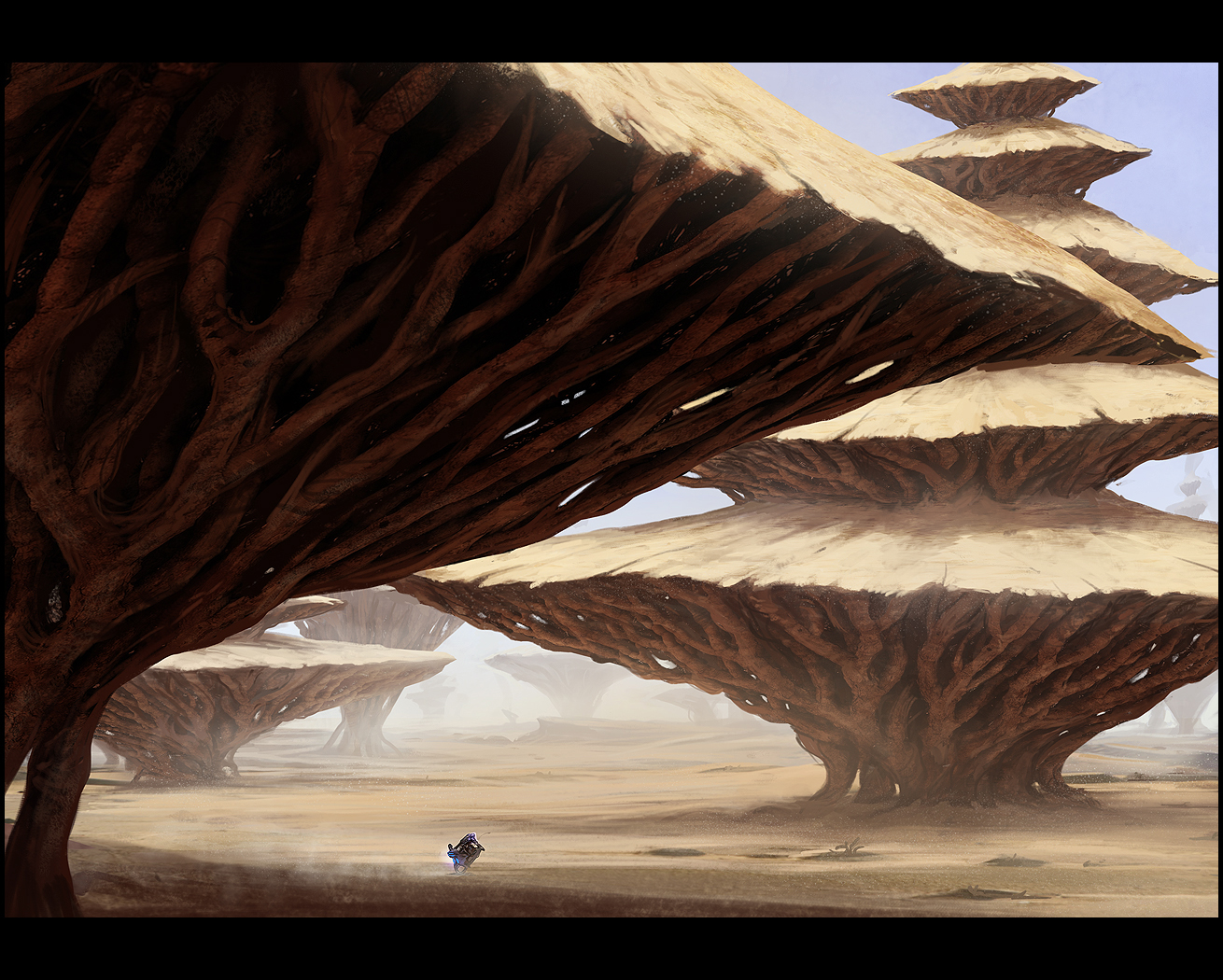The image is an illustrated, sci-fi desert landscape showcasing unique tree-like structures. On the left side, a tree structure with a small trunk leads to a broad, flat canopy composed of many tree trunks bundled together and topped with a brown hay-like layer. On the right, similar structures are tiered, with each level narrowing at the base and widening at the top, stacked three to five times, forming mushroom shapes that grow progressively smaller upwards. The background features a blue sky with a dust-filled, barren desert scene. A small dark object, possibly a person, is barely visible at the bottom left, emphasizing the immense scale of these intriguing, otherworldly trees.